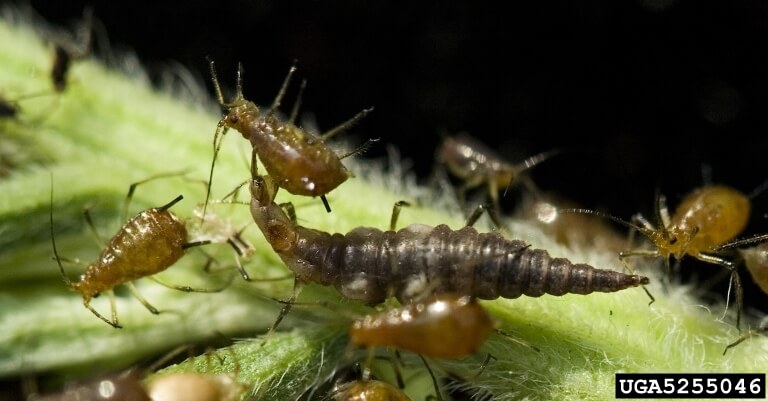In this detailed, zoomed-in image, we observe a scene on a green, hairy plant in a very dark background, possibly taken in a controlled environment. At the center, there's a large, black insect with a prominent abdomen, seemingly engaged in a conflict with numerous smaller, rounded, yellow insects that resemble ticks or ants. The larger insect appears to be gripping one of the smaller insects with its mouth. The finer details of the plant, including its tiny white hairs, are in sharp focus. On the bottom right corner of the image, the identifier "UGA 5255046" is clearly visible in white text against a black background.